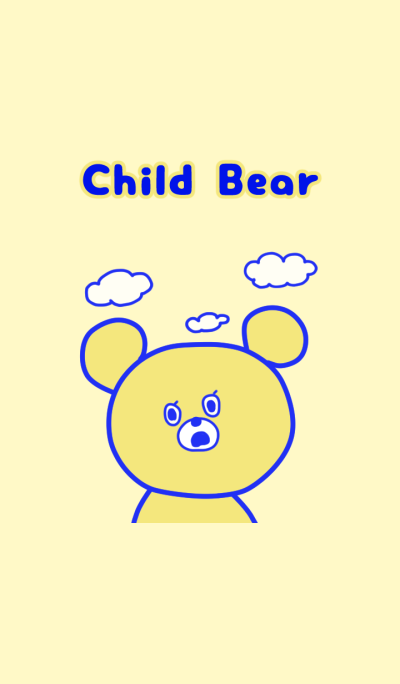The image features a cartoon drawing of a bear set against a light creamy yellow background, with visual elements suggesting it might be suitable for children's merchandise, such as a t-shirt or a phone wallpaper. At the top of the image, the blue text "Child Bear" is accented with a yellow border. The bear, with a blue outline, is centrally positioned and has a confused expression, looking directly at the viewer. The bear's face is yellow with unevenly round ears, white circular eyes with blue centers, and a white nose and mouth area featuring a black dot for the mouth and a blue dot for the nose. Above the bear's head float three white clouds with blue outlines, with the middle cloud being the smallest among them.